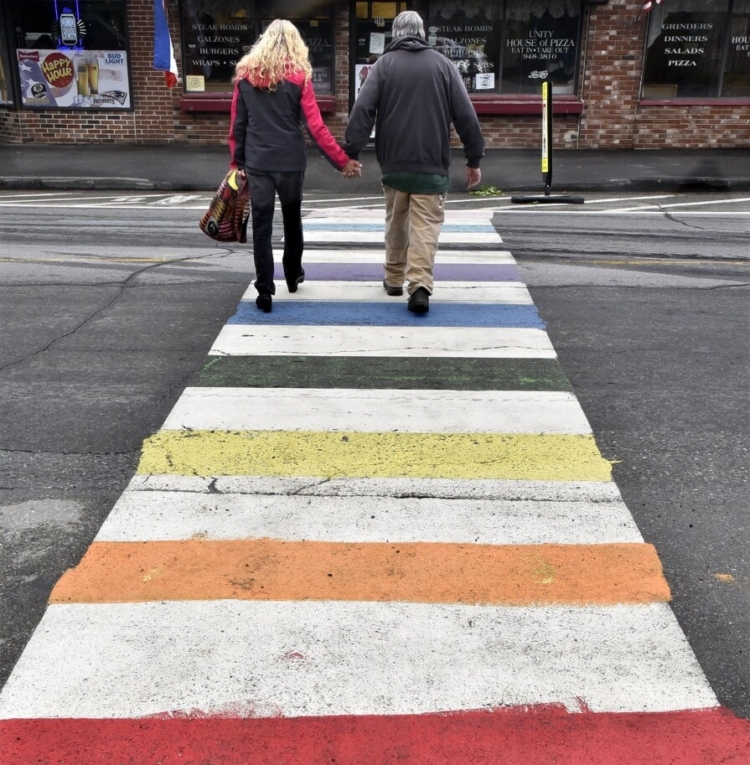This vibrant color photograph captures an older couple walking hand-in-hand across a crosswalk adorned with rainbow-colored stripes. From the bottom of the frame to about the top third, the crosswalk features alternating stripes of red, white, orange, white, yellow, white, dark green, white, blue, white, lavender, white, an unpainted section, white, and light blue. The couple is about halfway across, with the woman on the left and the man on the right.

The woman has long, blonde curly hair and is wearing black pants and a black jacket with a red stripe across the top. She holds a large reddish bag in her left hand. The man has silvery hair and wears beige pants, black boots, a gray sweater, and a green shirt that peeks out from under his sweater.

On either side of the crosswalk, the dark asphalt shows signs of wear, particularly on the left side where it's slightly cracked. The far side of the crosswalk features a set of angled stripes before transitioning into a dark paved sidewalk. Behind this sidewalk lies a brick wall with dark windows. Some windows in the center have a red line beneath them and display white text that advertises various businesses, including happy hour specials.

The couple is crossing in front of a storefront that appears to be a pizza shop named "Unity House of Pizza," as indicated by the visible signage. The photograph gives a sense of the urban environment, focusing on the couple making their way across the vividly painted crosswalk.